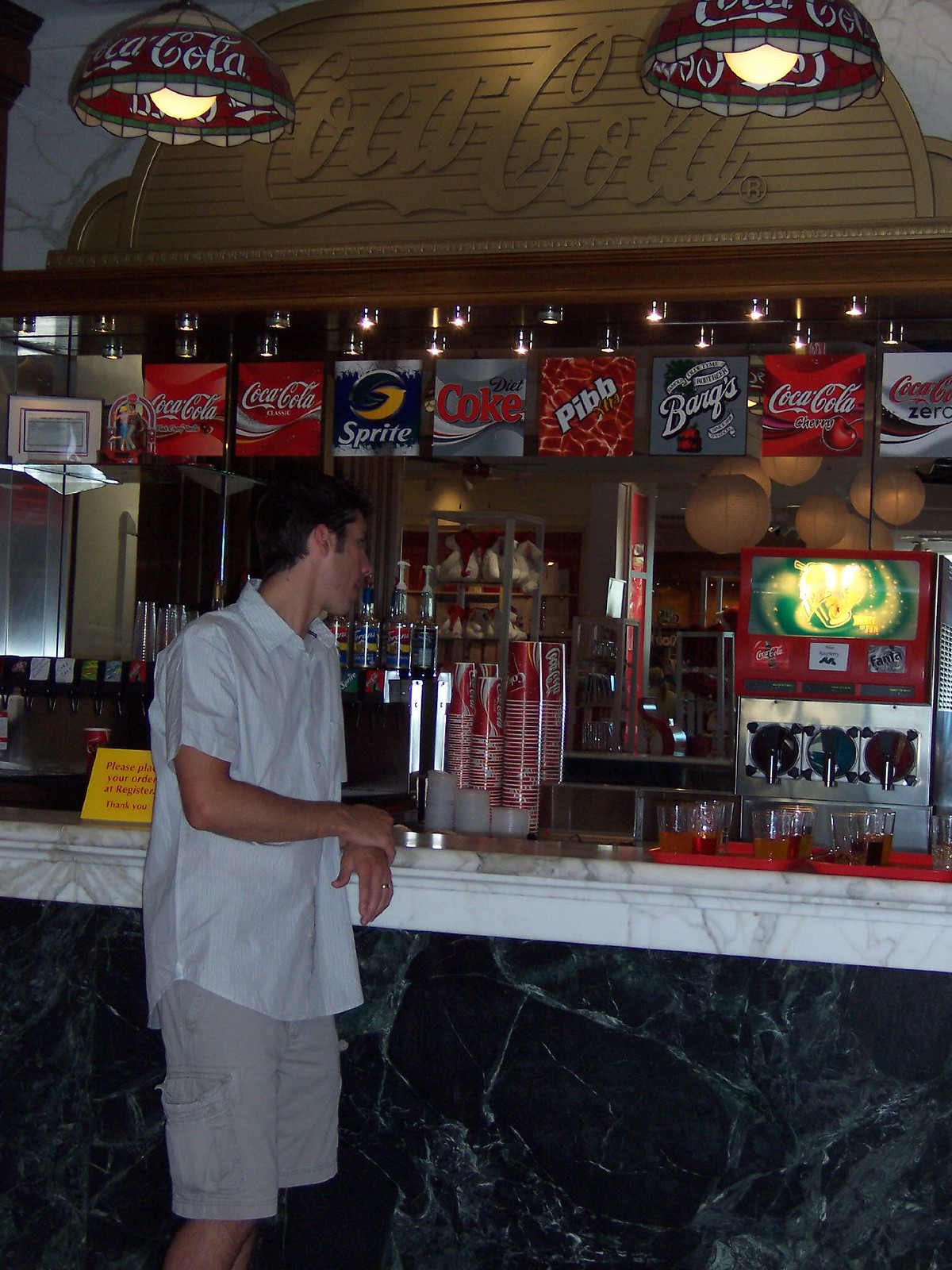In the image, a young white male with tannish pale skin and dark hair stands at a marble countertop inside a Coca-Cola-themed concessions stand. He wears an oversized, short-sleeved, collared white shirt and tan khaki cargo shorts. The countertop features a darker grayish-black base and a white rim, with a yellow sign reading "Please place your order at register thank you." Above him, two stained glass lamps with red and white Coca-Cola designs hang from the ceiling, illuminating the scene.

The backdrop includes an array of drink taps labeled with various Coca-Cola products such as Coca-Cola, Sprite, Diet Coke, Mr. Pibb, Barq's Root Beer, and Coca-Cola Zero. To the right, a soda machine is visible, along with a slushie machine that offers Coca-Cola and Fanta slushies. There are several red trays with half-filled glasses of beverages and stacks of Coca-Cola cups on the counter. The atmosphere is reminiscent of an old-time soda fountain, underscored by the multiple Coca-Cola banners and signs adorning the area. The young man appears to be in the process of placing an order, as he leans against the marble counter.